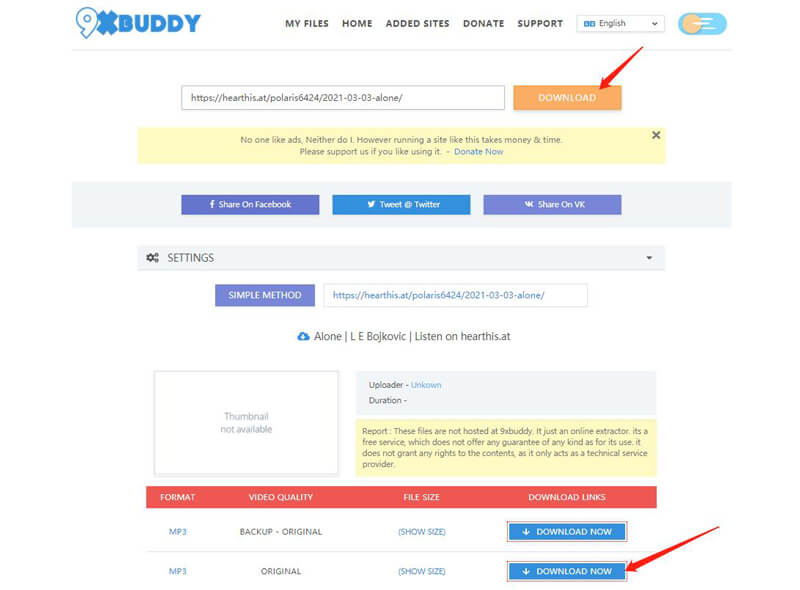**Website Overview: 9xbuddy**

The 9xbuddy website features a blue-themed logo with the number '9' displayed in white font and a blue outline. At the top of the homepage, there are several navigation tabs, including My Files, Home, Edit Sites, Donate, and Support, as well as a language switcher currently set to English.

Central to the page is an input area where users can paste a link, accompanied by an orange 'Download' button with a red arrow pointing to it for emphasis. Below this section, a yellow box states, "No one likes ads, and neither do I. However, running a site like this takes money and time. Please support us if you like using it," followed by a blue 'Donate Now' link.

Further down, there are social media buttons for sharing content on Facebook, Twitter, and VK. The page also includes a settings section, a blue button labeled 'Simple Method,' and another area for pasting a link.

A thumbnail area displays a box with the text "Thumbnail Not Available." To the right, there is information about the uploader, marked as 'Unknown,' and the video's duration also listed as 'Unknown.' Lastly, several mp3 files are available for download, each within blue boxes labeled 'Download Now,' with options for 'Backup Original' and 'Original.'